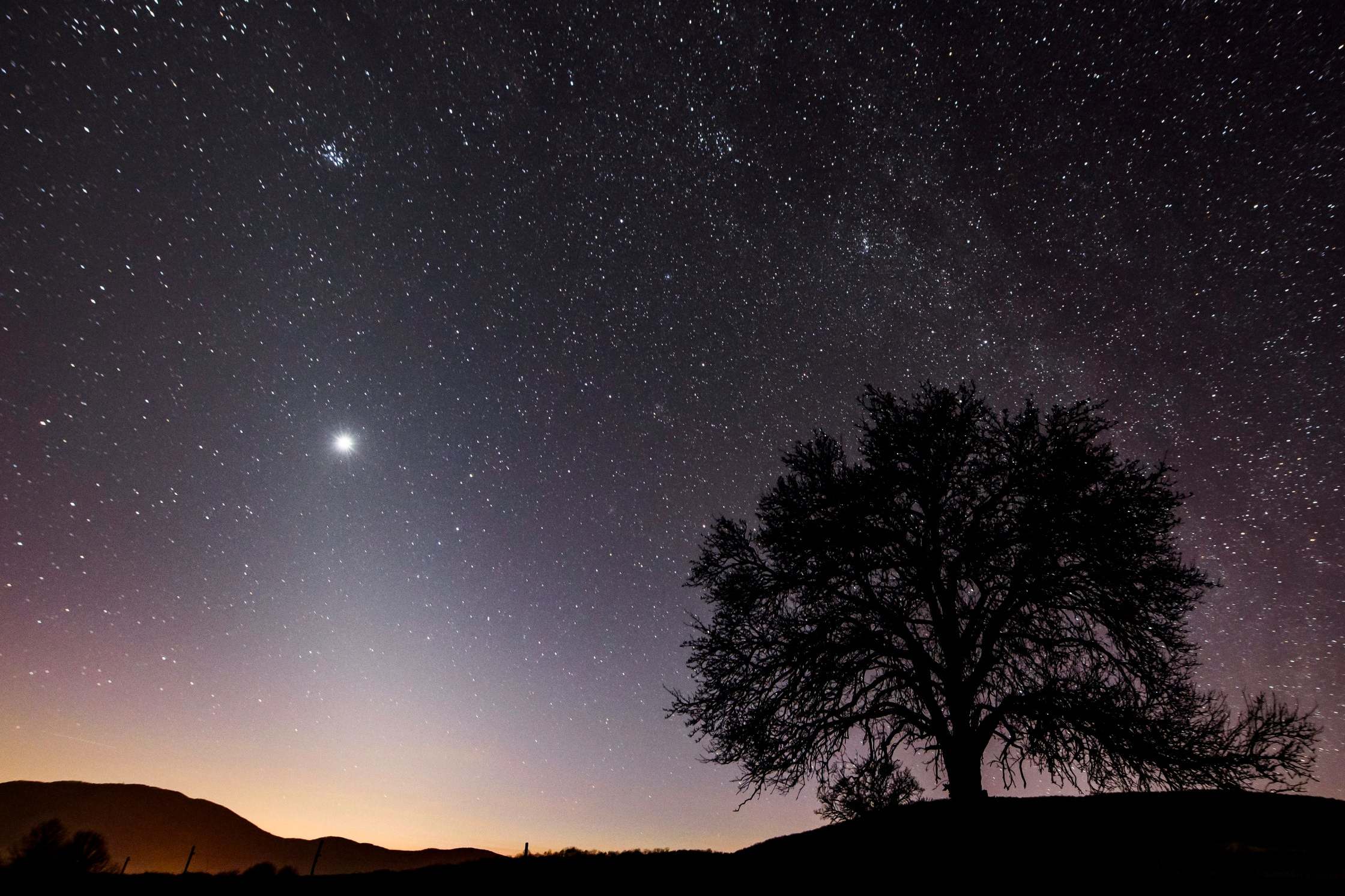This nighttime photograph captures a mesmerizing landscape with a star-filled sky, revealing intricate details as you look closer. Dominating the right side of the image is the silhouette of a large tree with sprawling branches that extend all the way to the ground, shrouded in darkness. The silhouetted tree appears black against the diverse hues of the night sky. The slightly hilly terrain forms the base of the photograph, occupying roughly the bottom 10% of the frame, also enshrouded in darkness such that no details can be discerned.

The night sky above the valley is a captivating gradient, transitioning from a light yellowish-orange haze near the horizon to a nearly black hue at the top, passing through layers of dark blue and purple. Scattered throughout the sky are countless pinprick stars, creating a dense, star-studded canopy. One particularly bright point of interest, positioned slightly to the left of the center, shines radiantly, almost as though it’s projecting light onto the Earth below. This brilliant star stands out against its smaller counterparts, adding a focal point in the beautiful celestial display.